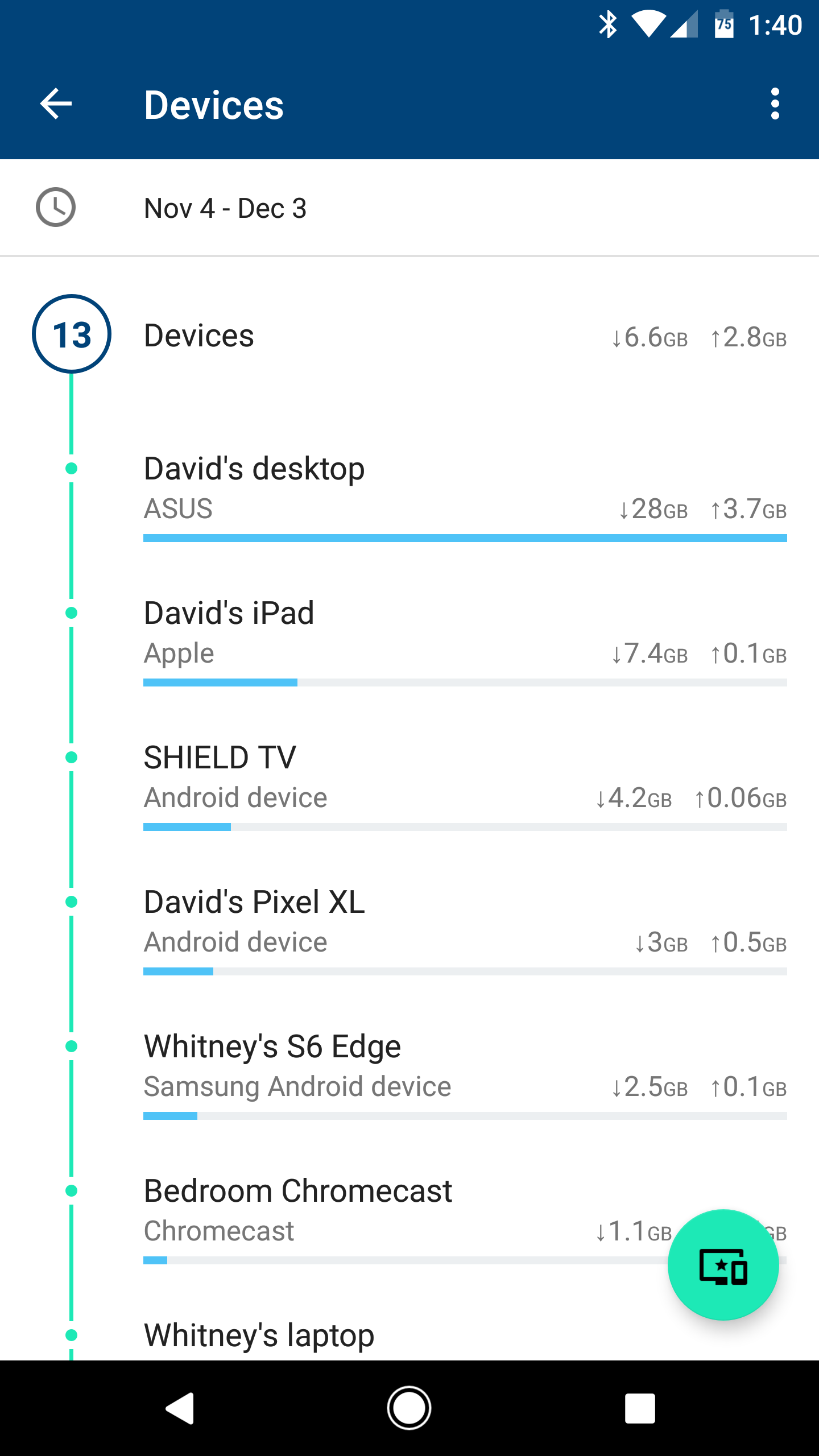This is a detailed description of a screenshot from an Android app, likely displaying data usage statistics from November 4th to December 3rd. 

The screenshot shows a summary indicating that a total of 13 devices used 6.6 GB of data during this period. In addition, there's an upward arrow marking 2.8 GB and a downward arrow marking 6.6 GB, which likely represent upload and download usage, respectively. 

The devices are listed in descending order based on their data consumption:

1. **David's Desktop (ASUS)**: This device has consumed the most data.
2. **David's iPad (Apple)**: This device ranks second in data usage.
3. **Shield TV (Android device)**: This device comes next.
4. **David's Pixel XL (Android device)**: This device follows Shield TV.
5. **Whitney's S6 Edge (Samsung Android device)**: This device is subsequent.
6. **Bedroom Chromecast (Chromecast)**: This device comes after Whitney's S6 Edge.
7. **Whitney's Laptop**: This device follows the Bedroom Chromecast.

It can be inferred that there are more devices on the list, but they are not visible in the current view of the screenshot, indicating the page can be scrolled to see details about the remaining devices. 

Additional details in the screenshot include a medium-level battery icon and a connection status that appears average, suggesting the user took the screenshot from an Android device, as the interface is not identifiable as that of an iPhone.